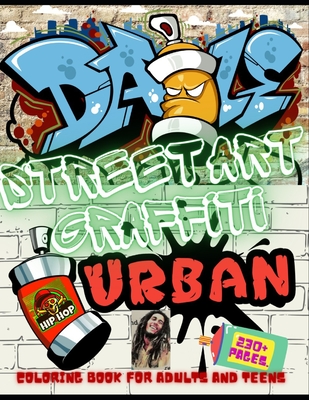The illustrated book cover features a vibrant street graffiti style, dominated by shades of blue, gold, green, and red. At the top, the background showcases a cityscape silhouette against a teal sky, overlaid with various graffiti fonts. The largest graffiti text reads "D-A-I-L-E," where the 'I' is stylized as an orange character with white eyes. Scattered among the graffiti are the words “Days,” “Street Art,” “Graffiti,” and “Urban.” 

Central to the cover, a green text outlined in white spells out "Street Tart Graffiti," and a bold red text with black outlines at the bottom reads, “Coloring Book for Adults and Teens, 230 plus pages.” A photograph of a smiling man with long dreadlocks—resembling Bob Marley—is positioned under the ‘R’ of "Urban." Nearby, there's an illustrated spray paint can labeled "Hip Hop," featuring a menacing skull with red glaring eyes. The background appears to be a white brick wall, adding to the urban aesthetic. This high-energy, cluttered design encapsulates the chaotic yet artistic essence of street culture.